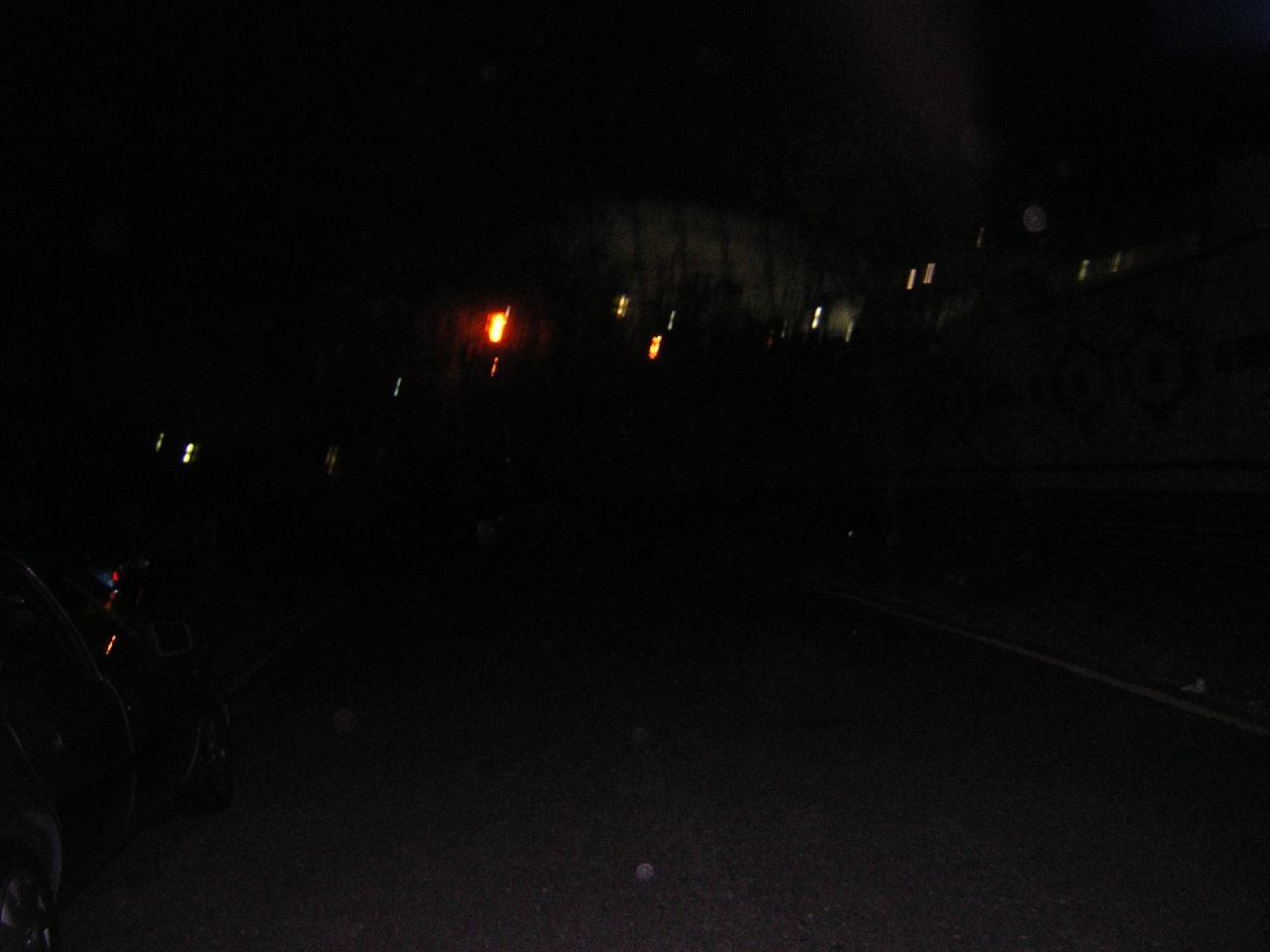This is a nighttime photograph captured from the left side of a road or parking lot. The scene is predominantly dark, with the limited range of a flash highlighting only a small portion of a nearby car on the left side. The image is mostly enveloped in deep black shadows, conveying an eerie and almost mysterious atmosphere. In the distance at the vanishing point, a bright yellow light—possibly a streetlight or stoplight—punctuates the darkness. Scattered around this light, small white or silver rectangles, likely reflectors, glimmer faintly. Further in the background, there is a lighter patch of color, hinting at the presence of a building or a sign. On the right-hand side of the photograph, a bit of wall is visible, adorned with a circular pattern featuring dots in the center. Despite the overall obscurity, these subtle elements offer intriguing hints of the surrounding environment.